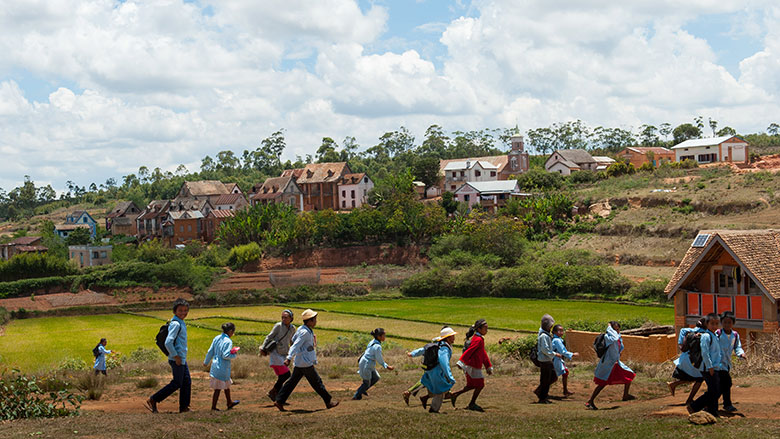The photograph captures a lively scene of children, likely from a rural village in South America, walking and skipping energetically along a dirt path. The children, who appear to be of various age groups but similar in age, are all clad in school uniforms consisting of light blue shirts, with some girls wearing red skirts or dresses. Many are equipped with backpacks and a few don hats or other outerwear. They walk against a picturesque backdrop featuring a verdant, grassy field and a series of traditional village houses that climb up along terraced, hilly terrain. The houses give way to lush greenery and trees, under a bright blue sky filled with fluffy white clouds, contributing to the vibrant and sunny atmosphere of the scene.